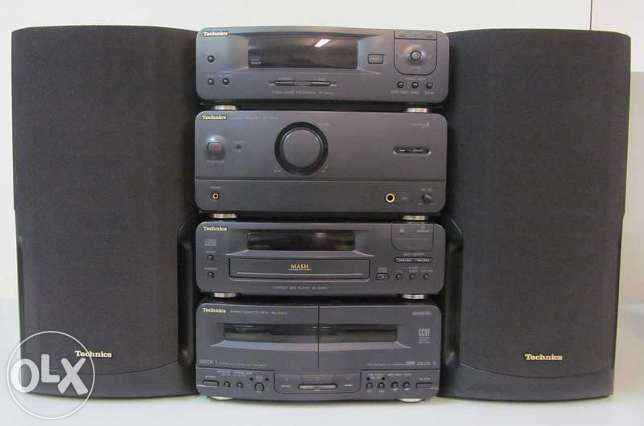This is a detailed photograph of an old stereo and speaker system. The setup features four music players stacked vertically in the center, flanked by two large, dark grey (perhaps black) Technics brand speakers on either side. The word "Technics" is inscribed in gold at the bottom of each speaker. The entire system stands against a white wall and is positioned on a white table.

The topmost player has a shiny, reflective panel and bears the Technics brand name at the top left corner. To the right, beneath a small panel, there are three buttons whose labels are unclear due to the photo's slight blurriness. Below this is a unit with a central knob, flanked by what appear to be headphone and electrical jacks at its base.

The third unit down resembles a video cassette player with a long slot likely for VHS tapes, accompanied by a black reflective strip above it. The bottom player is likely a tape deck, identified by a vertical seam down the center for tape insertion and multiple buttons at the bottom left and right.

In the lower-left corner of the image, a watermark in the form of a white circle with the letters "OLX" is visible. The photograph is square-shaped, ensuring all elements are clearly centered and framed within the shot.